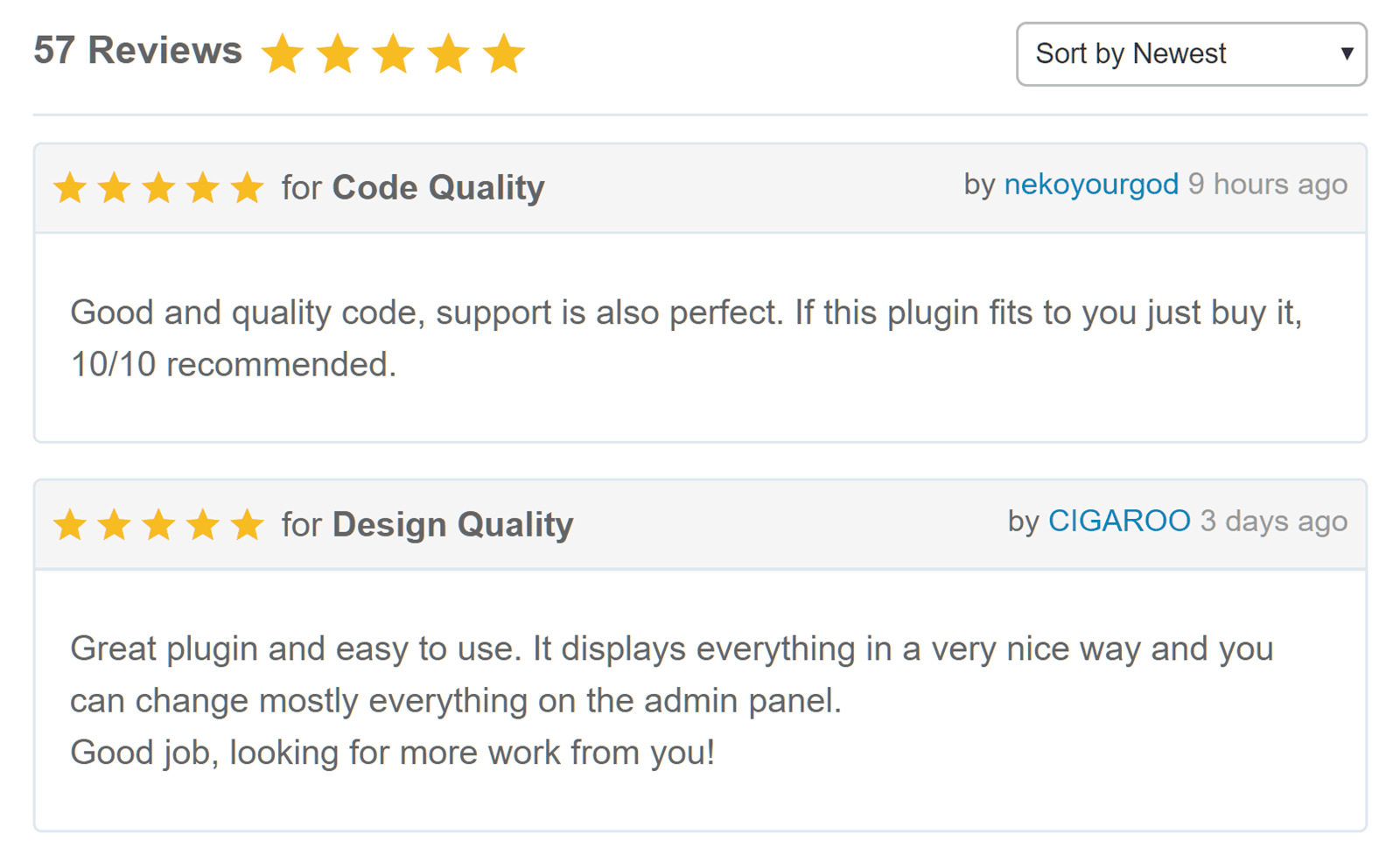The image captures a screenshot showcasing two distinct product reviews. At the top-left corner, there's an indicator showing "57 reviews" accompanied by five orange-yellow stars symbolizing the average rating. On the right side, there's a drop-down menu box labeled "Sort by newest."

The first review emphasizes code quality, marked with a 5-star rating. The review text praises the plugin for its good quality code and perfect support, with a strong endorsement: "If this plugin fits you, just buy it, 10 out of 10 recommend." This review was written by a user named Neko Your God, 9 hours prior to the screenshot.

The second review also features a 5-star rating, this time highlighting design quality. Written by a user named Siguru 3 days ago, the review commends the plugin as being great and easy to use, noting that it displays everything clearly and allows for extensive customization, ending with a "good job."